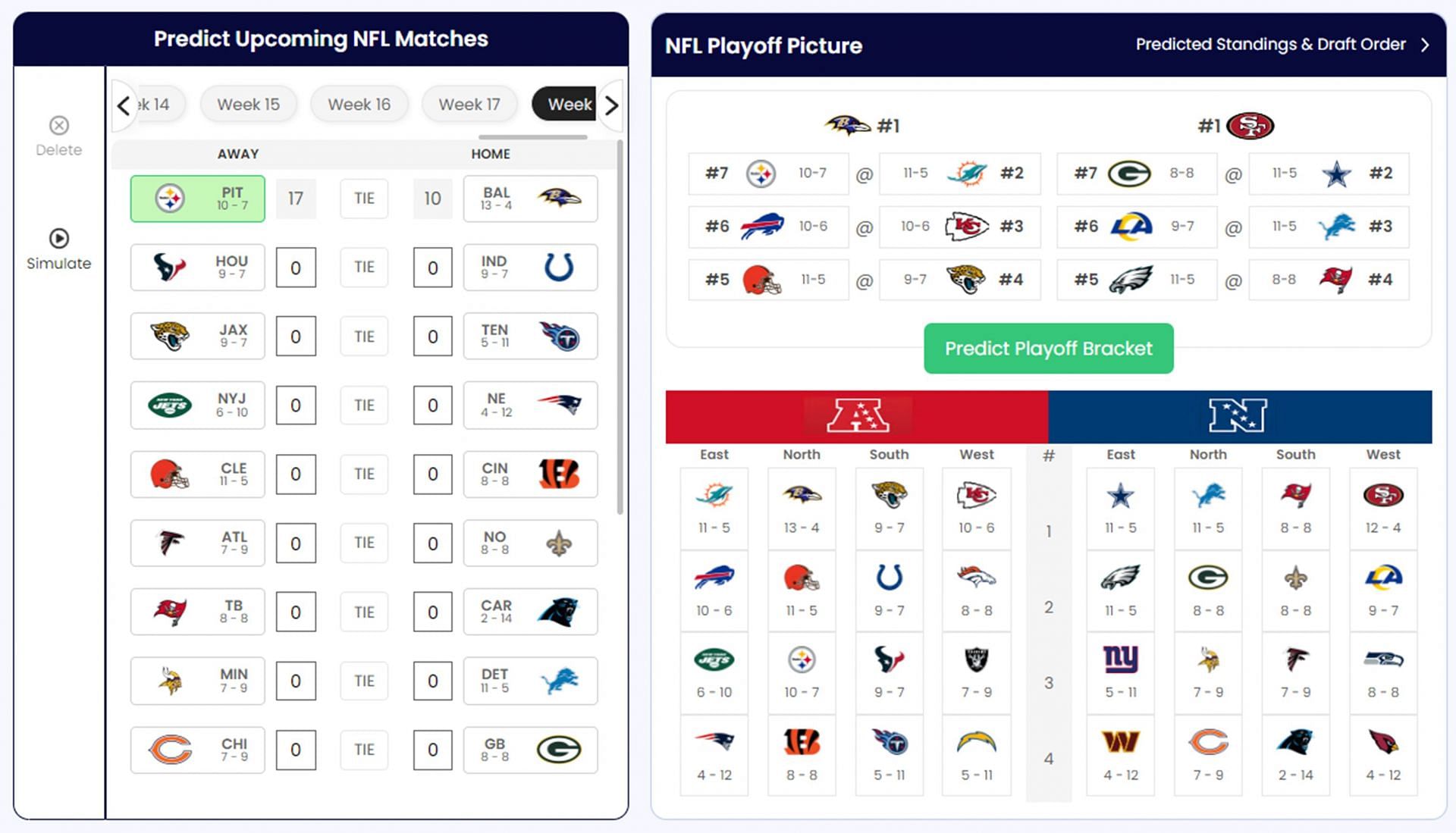This image appears to be a comprehensive dashboard from a sports website dedicated to NFL football. The main interface highlights several key features for predicting and simulating upcoming NFL matches. At the top, a prominent header reads "Predict Upcoming NFL Matches," with various weeks available for selection. Functional buttons like "Delete" and "Simulate Certain Matches" are visible, allowing users to manage predictions.

The layout includes two distinct sections. The left section features match predictions, displaying icons of sports teams, likely NFL teams, along with their scores, wins, and losses. Each match showcases the home and away teams, with their respective logos and stats.

On the right side, a more horizontal section presents an "NFL Playoff Picture," which includes predicted standings and draft order. Teams are listed with their prospective placements, ranging from first place to fourth place, and possibly beyond. Additionally, a "Predict Playoff Bracket" tool is located at the bottom, which enables users to simulate playoff outcomes.

The interface is enhanced with colorful icons, such as a red "A" and a blue "N" with stars, likely representing different prediction options or tools, though their exact functions are unclear. Overall, the website offers a robust platform for NFL enthusiasts to engage in match predictions and tracking team standings throughout the season.